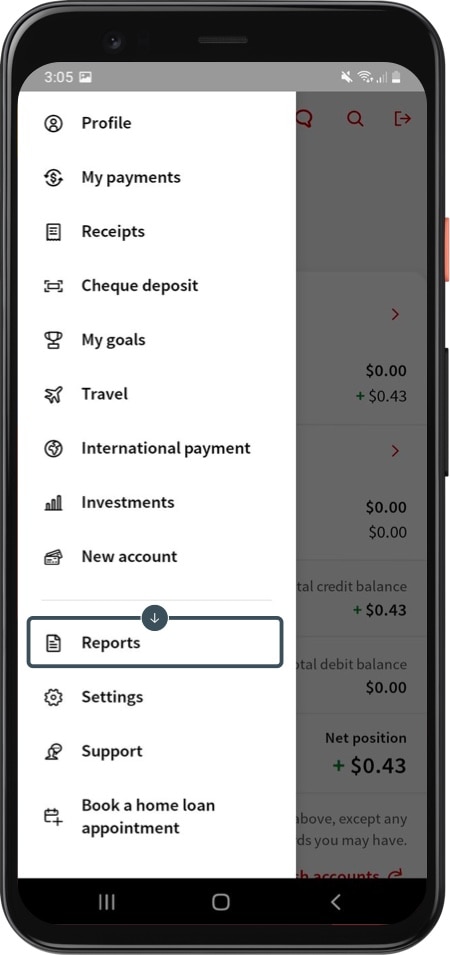The image depicts a mobile phone in a black case, showcasing its left side with clearly visible red power and volume buttons. The phone's screen displays a bank's profile section window, which overlays the original page, graying out the background. The profile window contains a list of options: "Profile," "My Payments," "Receipts," "Check Deposit," "My Goals," "Travel," "International Payment," "Investment," and "New Account" at the top. Below these, there's another section titled "Reports," highlighted in a black box with a down arrow in the middle. Further options include "Settings," "Support," and "Book a Home Loan Appointment," each accompanied by its respective icon. The phone's camera is also visible at the top left corner of the case.